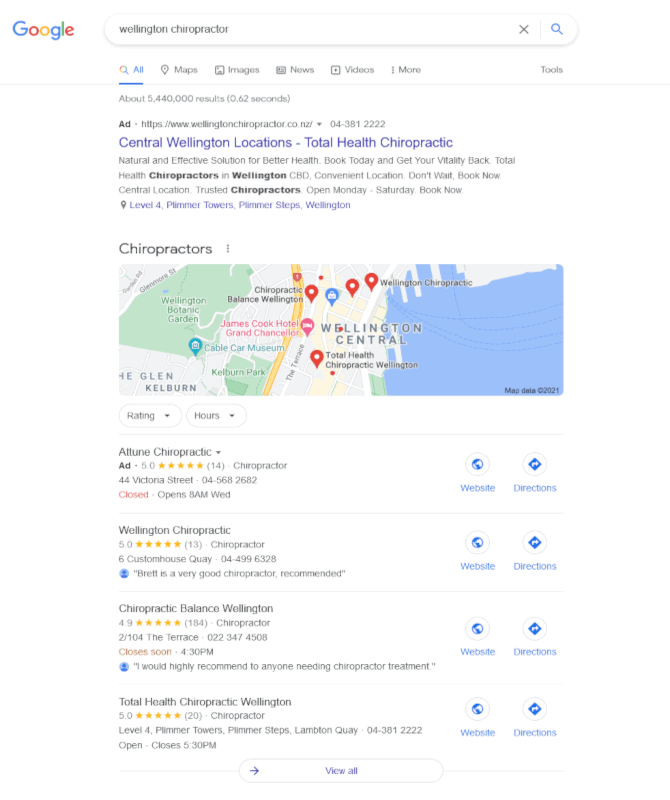The image depicts a Google search results page on a desktop. The search query entered is "Wellington chiropractor," returning approximately 5,440,000 results. At the top, there is an advertisement for "Central Wellington Locations - Total Health Chiropractic."

Beneath the ads, the standard Google Maps result appears, showing key locations like Wellington Botanical Gardens, James Cook Hotel, and some water bodies, indicative of the typical Google Map interface. 

The detailed list starts with an ad for "Attune Chiropractic," which boasts a five-star rating based on 14 reviews. The listing provides options to visit the website or get directions. 

Next is "Wellington Chiropractic," also with a five-star rating from 13 reviews. It's located at 6 Customhouse Quay with a contact number of 044996328. A featured review quotes, "Brad is a very good chiropractor, recommended."

Following is "Chiropractic Balance, Wellington," with an impressive rating of 4.9 stars from 184 reviews. The clinic is situated at 2/104 The Terrace and closes soon at 4 p.m. It comes highly recommended for those in need of chiropractic treatment.

The last entry is for "Total Health Chiropractic, Wellington," which holds a perfect five-star rating from 20 reviews. It is located on Level 4 of the Front Towers and remains open until 5:30 p.m. 

At the bottom of the listing is an option to "View All" for more results.